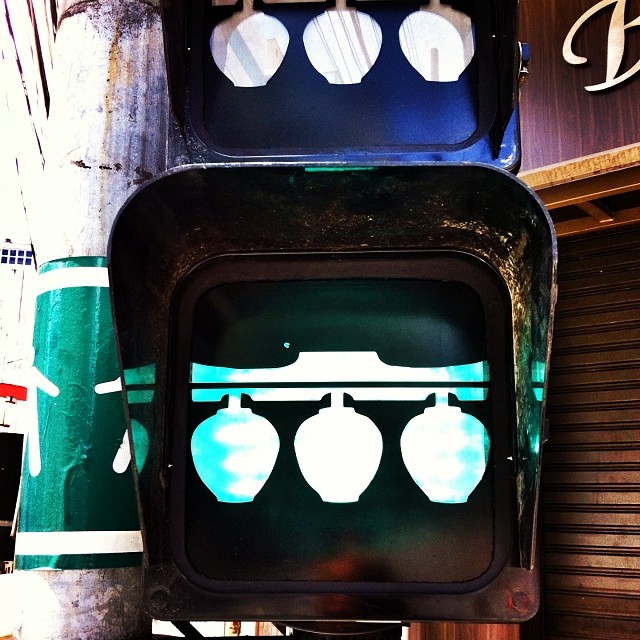This photograph captures an unconventional and intriguing traffic signal mounted on a post. The focal point of the image showcases a signal device that diverges from the typical traffic lights, boasting three spherical objects hanging horizontally from a yoke-like structure, akin to hornets' nests or perhaps vases. These spheres are currently unlit, leaving the colors – potentially red, yellow, or green – indiscernible. The post to the left features a green sticker displaying a simplistic stick figure, likely indicating a pedestrian walkway.

To the right of the signal, there is a corrugated metal shutter, characteristic of a closed shop door, adding to the urban setting. The background includes another metal object, possibly green in color, though its purpose remains ambiguous. The store in the upper right corner has a sign starting with an elegant cursive 'B', but the rest of the name is obscured. Overall, the image presents a mysterious and non-standard traffic control device set against a backdrop of urban elements.